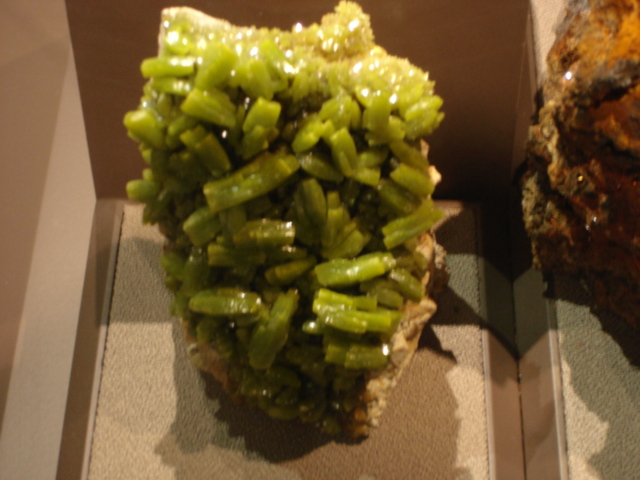The image portrays an up-close photograph of a modern art sculpture resembling a cluster of green crystals or green pepper-like structures fused together. The main green formation, reminiscent of small green beans or thin green pepper segments, exhibits a light green color akin to that of broccoli and is composed of numerous rectangular segments. These segments are rounded at the top and glisten under the light, creating a shiny effect. The base of the green structure appears beige and somewhat dirty, possibly showing the exterior of the material it's crafted from. 

The sculpture is set against a beige background that has a texture similar to Berber carpet, adding to the overall neutral, earthy tone of the scene. On the far right, there's a smaller adjacent figure, a darker rusty or brownish-orange toned object that appears to be made of plastic or adorned with fake jewels, adding contrast to the image. The entire composition rests on a light tan surface, completing the photograph's setting.